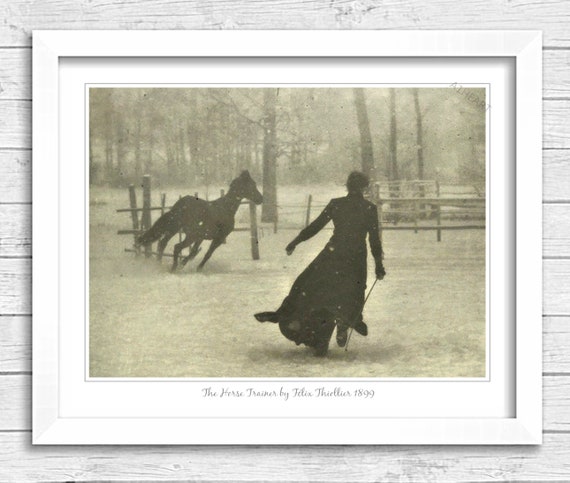This is a detailed image of a photograph encased in a white frame with a white matted inlay, placed on a light gray wooden background. The photograph, captured in black and white, appears to be from the late 1800s, specifically dated 1899. It features a scene of a person, possibly a woman, wearing a long, flowing coat or dress, running alongside a horse in a snowy yard. The backdrop reveals barren trees and wooden fence posts. The frame is captioned "The Horse Trainer" with the name "Felix Thelis" inscribed below. This elegant setup presents a nostalgic glimpse into a wintry day from the past.